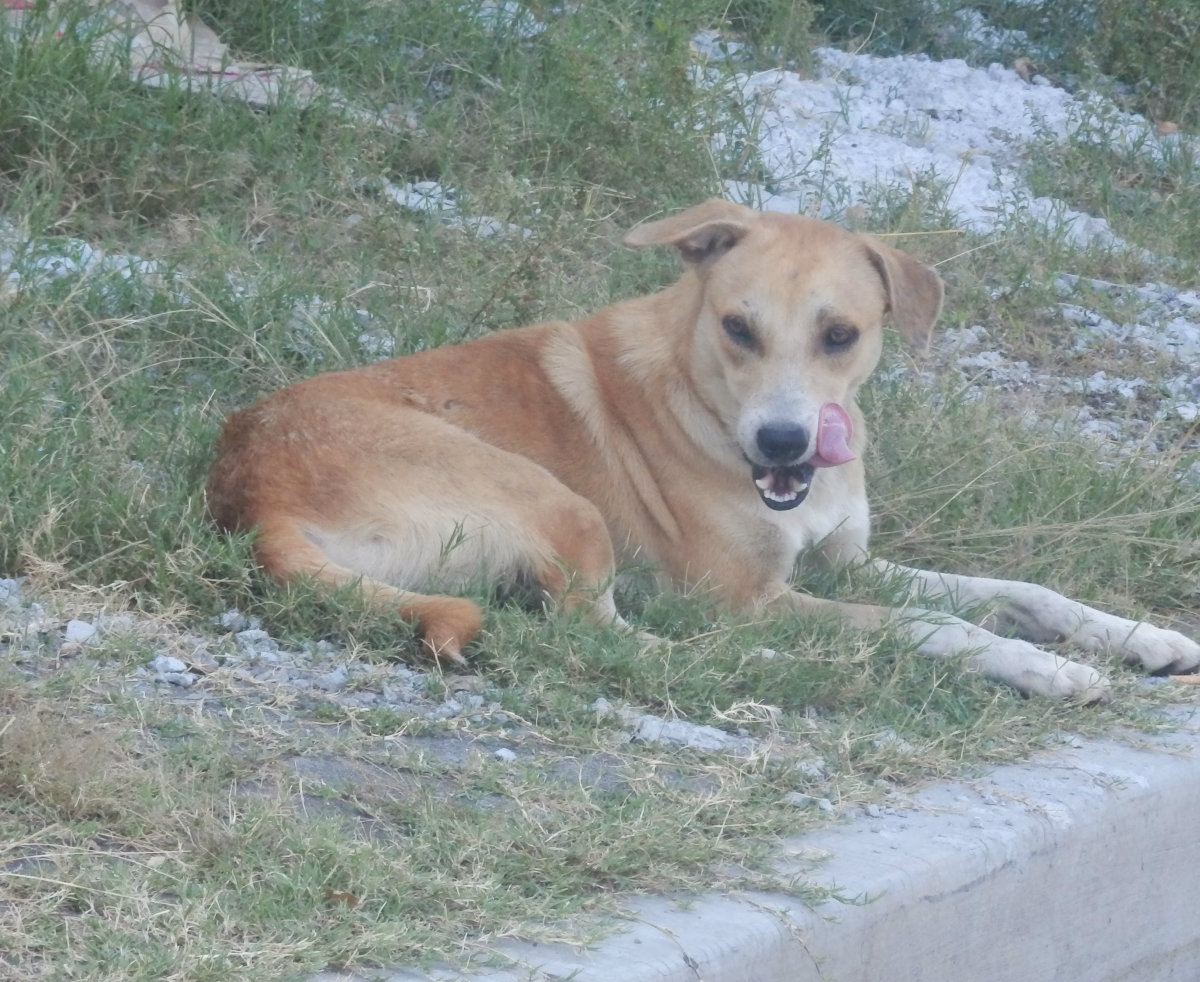This rectangular photograph, slightly wider than it is tall, depicts an outdoor scene with a larger tan, short-haired dog, resembling a Labrador, comfortably laying on a sparsely grassy incline. The incline has patches of gray, rocky areas indicating it is not fully covered with grass and could benefit from landscaping. The dog appears alert and relaxed, its tongue visibly sticking out to the left side of its mouth, as if it has just licked its chops. Its two front paws are stretched out, and its long tail is laid along its body. The setting is beside a street curb, visible in the bottom right corner, contrasting with the natural surroundings. The background behind the dog features a grassy hill, some of which seem to have remnants of snow. The dog’s golden eyes, slightly averted from the camera, suggest a state of calm attentiveness.